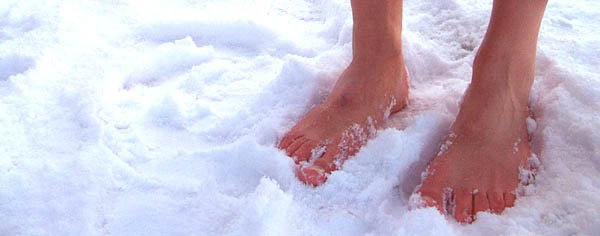The image depicts a stark winter scene featuring a pair of bare, frostbitten feet standing in the snow. The snow, around four inches thick, shows various prints and divots, indicating multiple previous disturbances. The feet, likely those of a teenager, are vividly red from frostbite, with snow clinging between the toes and piled up on one side. Only the lower legs up to six inches above the ankles are visible, revealing pale skin against the cold, white backdrop. The scene is accentuated by light reflecting off the snow from the sun in the top left corner, casting a cold, bright light over the pristine winter landscape.